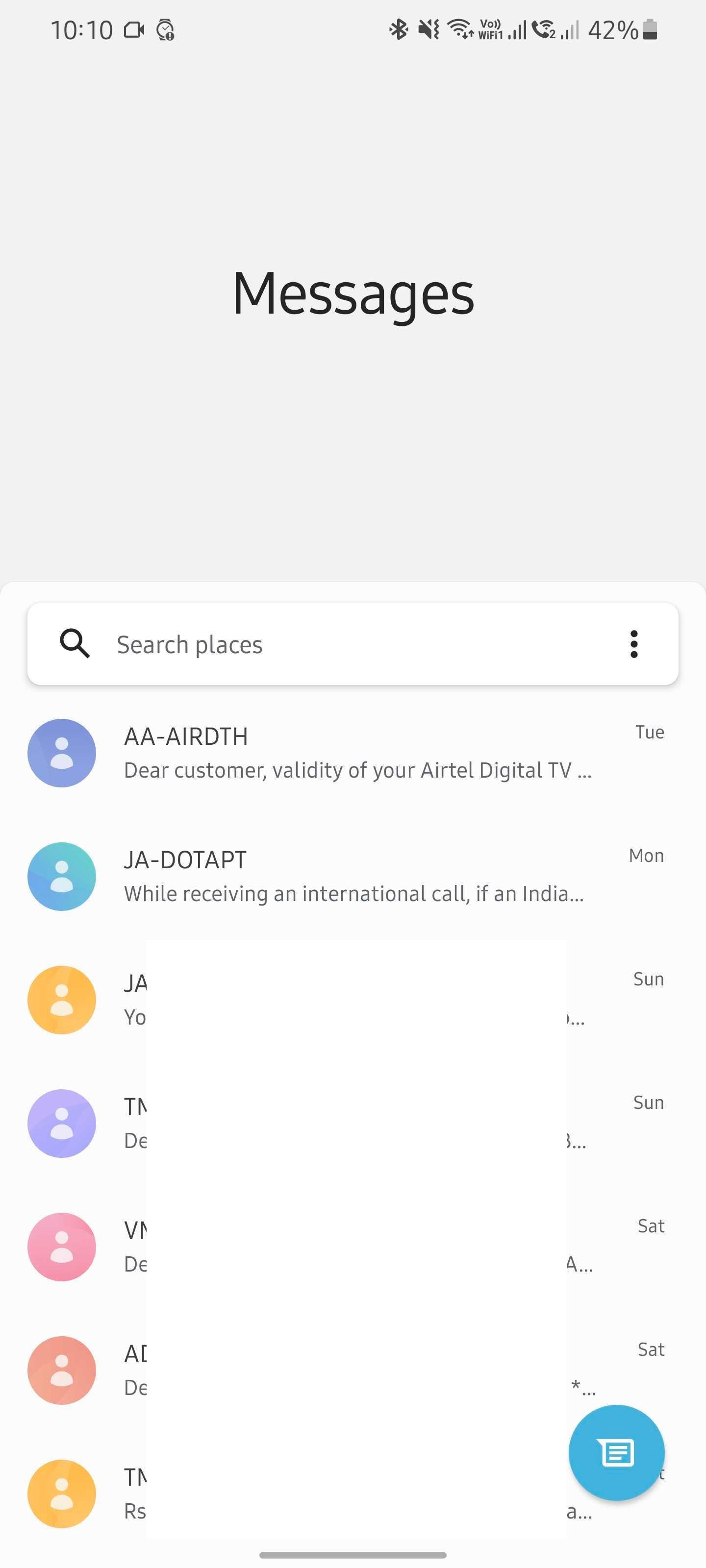The image captured on a phone screen displays a messaging app interface with intricate details. It features a large, light gray box prominently labeled "Messages" in black text. The top of the screen indicates a battery level of 42% and the current time, 10:10 AM, in the upper left corner, accompanied by several other status icons.

Beneath the primary gray box is a search bar labeled "Search places," which includes a search icon on the left and three vertical dots on the right for additional options. The first displayed message preview reads "AIRDTHT" and mentions the customer validity for Airtel digital TV, with further details accessible upon clicking. This particular message is linked to a generic blue person icon and is marked for Tuesday.

Additional message previews below are presented with varied colors and brief texts: 

- One from "JA.APT" with an interrupted message about receiving an international call if in India, accompanied by a teal icon.
- Several other message previews are partially obscured but feature unique profile icons in gold, purple, light pink, burnt orange, and another gold.

A noticeable blank pop-up obscures parts of the messages, showing only the dates they were sent: Sunday, Sunday, Saturday, Saturday. Finally, at the bottom of the screen, there is a prominent blue circular icon with a notepad symbol, indicating the option to compose a new message.